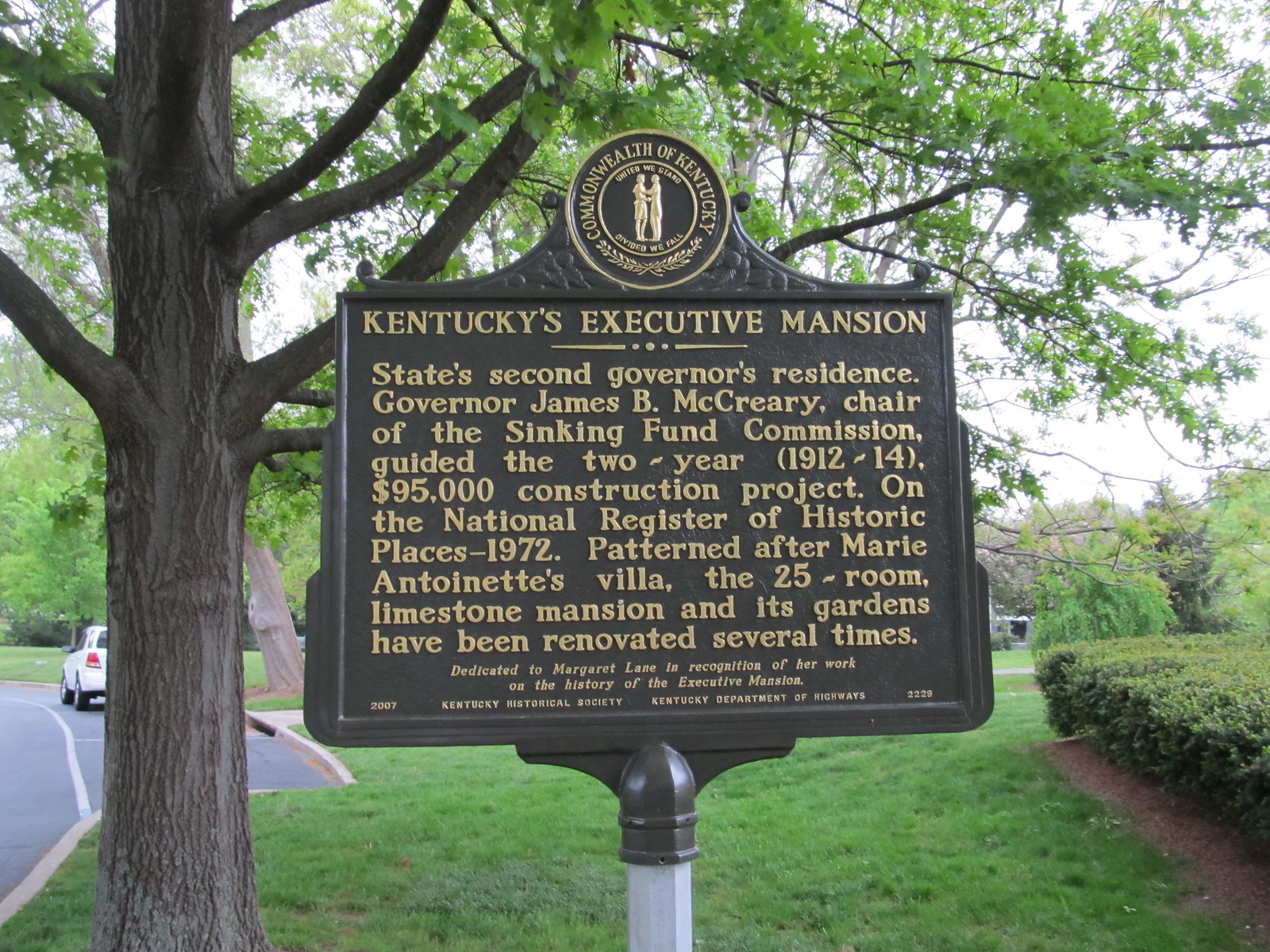This is an outdoor image of a metal sign mounted on a silver-gray metal pole. The sign itself is dark brown and features a distinctive circular emblem at the top with the gold text "Commonwealth of Kentucky" surrounding two figures standing next to each other. The sign reads: "Kentucky's Executive Mansion, State's Second Governor's Residence. Governor James B. McCreary, Chair of the Sinking Fund Commission, guided the two-year, 1912-14, $95,000 construction project on the National Register of Historic Places in 1972. Patterned after Marie Antoinette's villa, the 25-room limestone mansion and its gardens have been renovated several times." The background consists of lush greenery, including grass, trees, and hedges, giving it a serene, park-like setting. To the left of the image, there is a prominent tree trunk with branches and leaves, and a view of a parking lot area with a white car parked. The overall atmosphere is bright and spring-like, with overcast skies completing the scene.